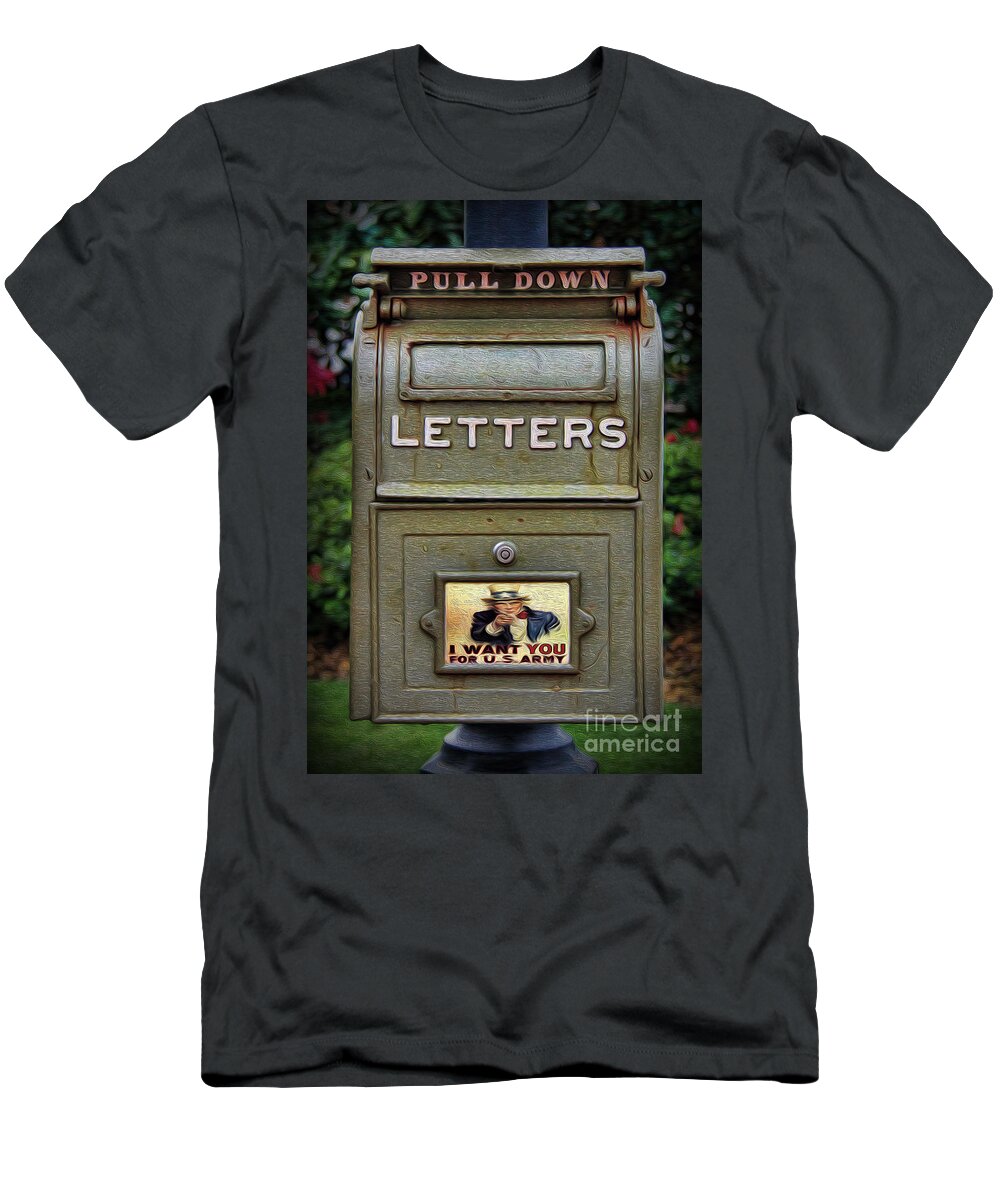This visually descriptive product photo showcases a black t-shirt laid casually against a white background. The shirt, slightly wrinkled but not crumpled, features a prominent image dominating its front. The image portrays an old-fashioned, olive-green mailbox affixed to a pole, accompanied by surrounding bushes and a few flowers, creating a garden-like setting. The mailbox bears the text "pull down" on the top and "letters" embossed below the mail slot. The bottom section of the mailbox integrates the iconic Uncle Sam poster, where a patriotic figure in a blue jacket and star-spangled top hat points directly at the viewer, emblazoned with the slogan "I want you for the U.S. Army" in bold red text. The picture has a dark vignette effect and is watermarked with "Fine Art America" in the bottom right corner, giving the entire image a professionally edited, Photoshop-like appearance.